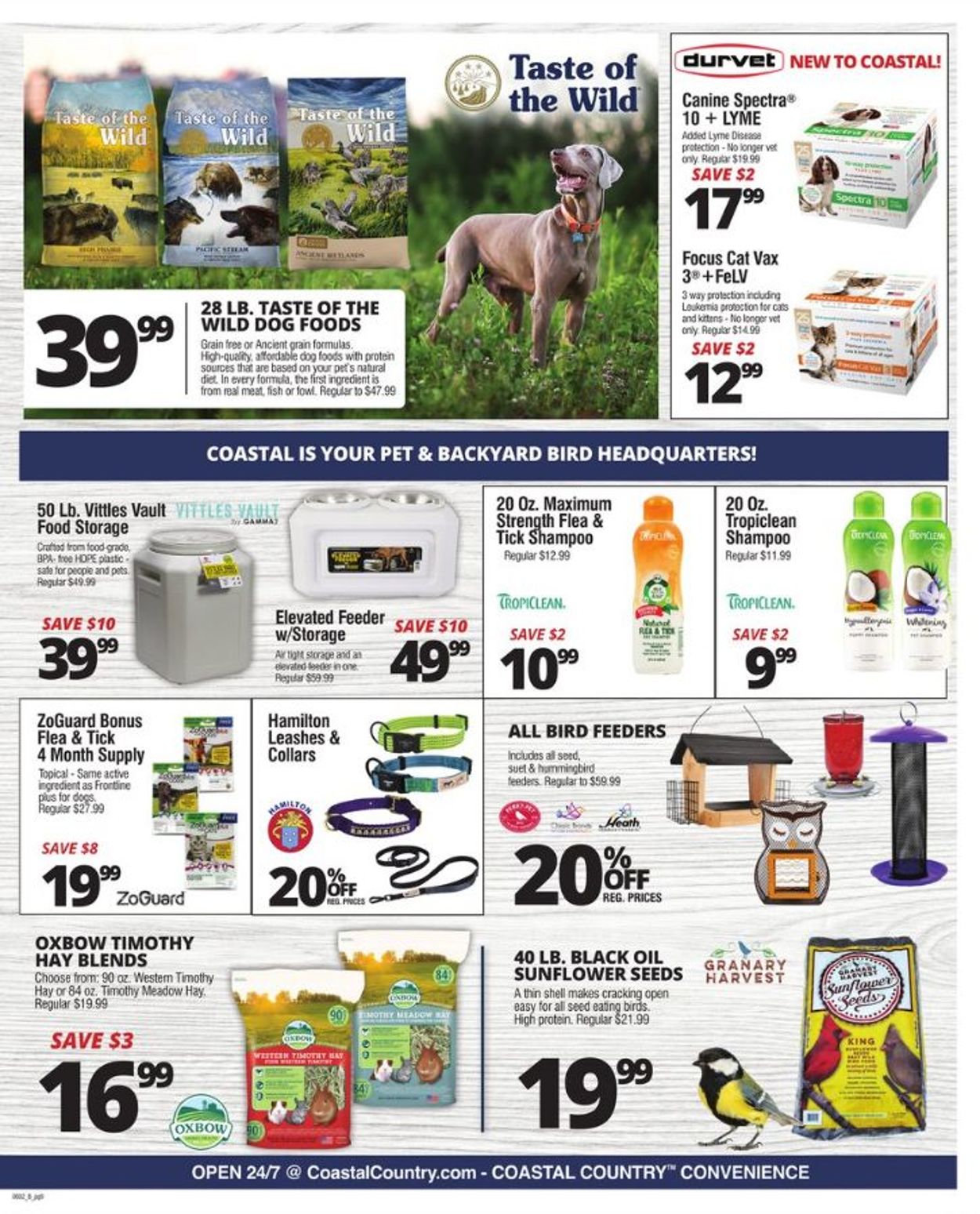This promotional flyer showcases an array of pet supplies. The top left corner features a prominent image of 28-pound bags of Taste of the Wild dog food, priced at $39.99 in large, bold text. Accompanying the dog food is a picture of a gray dog wearing an orange collar. Below this, there's an assortment of bird feeders. A significant text highlight reads "All bird feeders, 20% off regular prices," with the "20% off" emphasized. The bird feeders come in various designs, including a purple and black feeder, a red feeder, and an owl-shaped feeder. Adjacent to this section, the flyer advertises 40-pound bags of black oil sunflower seeds for $19.99, with the price displayed in larger text. A vibrant image features a yellow, black, and white bird, and another picture of the bird food shows a red bird and a gray bird. Finally, the flyer highlights a selection of leashes and collars, marked down by 20% off.